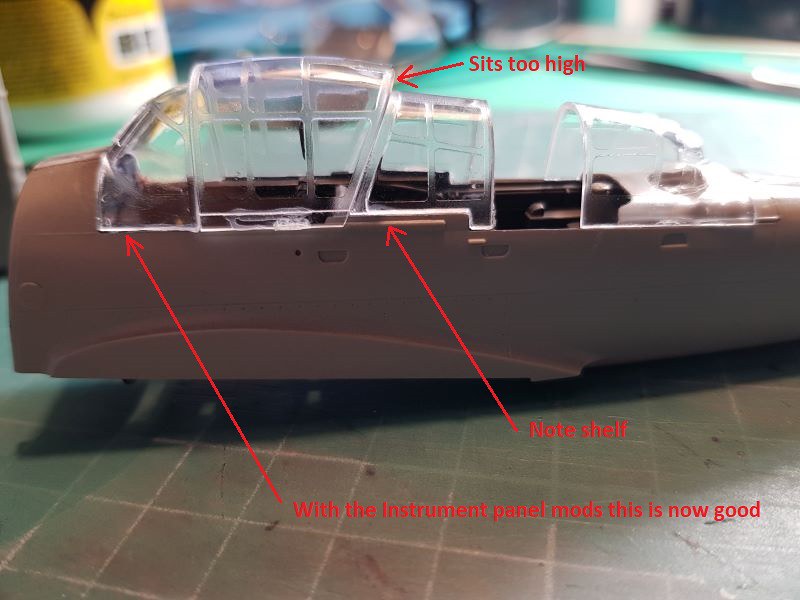The image is a color photograph of the fuselage of a model airplane, featuring several labeled red arrows and text. The fuselage, predominantly brown with patches of gray, is composed of plastic and includes clear, dome-shaped plastic on top, simulating a cockpit with cutouts where the wings would attach. A red arrow at the top points to the cockpit area with the text "sits too high." Another red arrow points to a small shelf next to the cockpit with the label "note shelf," and a final red arrow at the front reads "with the instrument panel mods this is now good." The fuselage rests on a surface with a grid pattern of small brown squares separated by white lines. The background is blurred but shows a teal wall and a yellow container with a white screen and black text.